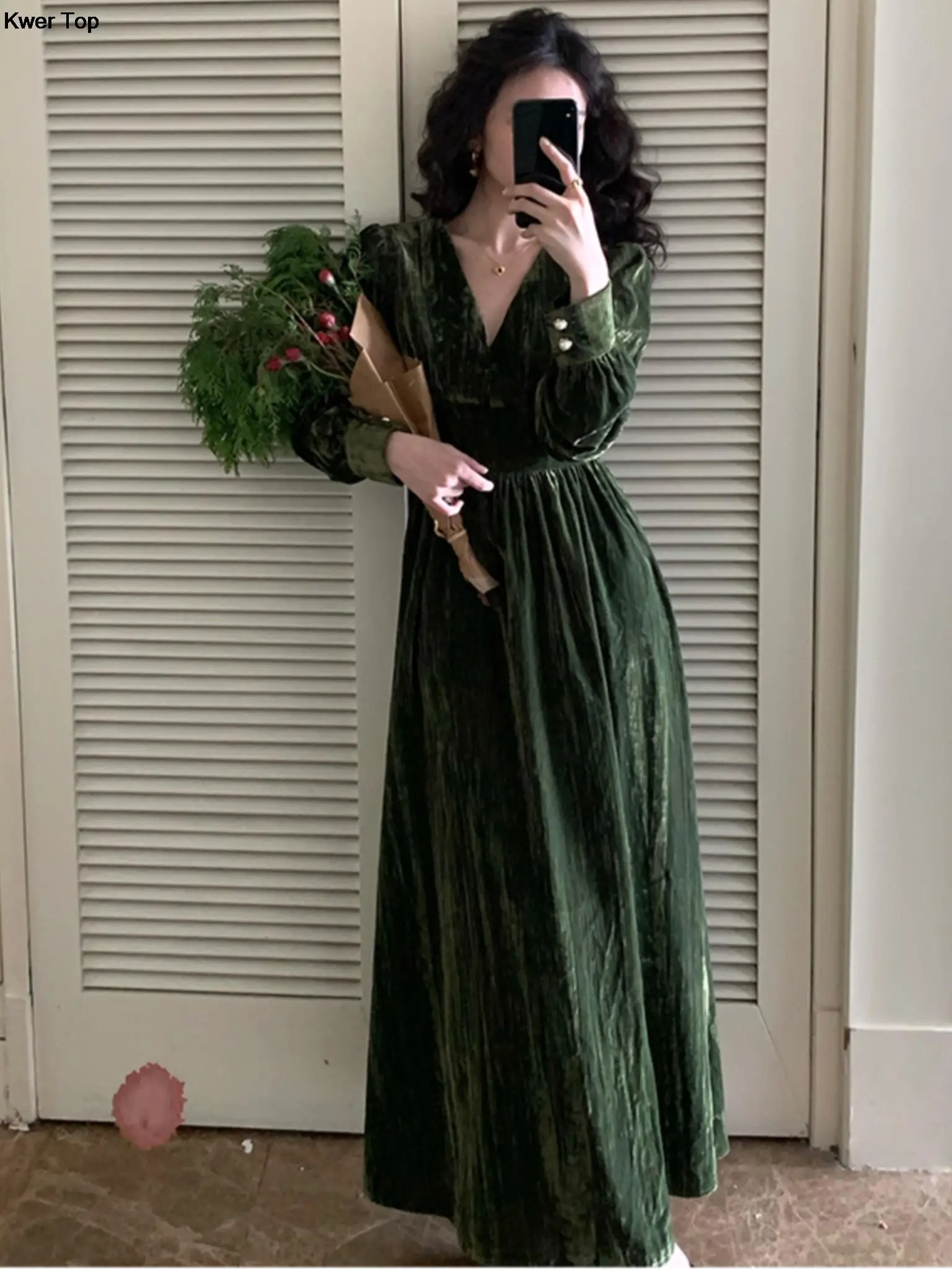The image captures a mirror selfie of a woman with long, dark hair, partially obscured by the black cell phone she is using to take the photo. She is wearing a dark forest green velvet dress with a V-neck, accented by small silver or gold buttons on the cuffs of her sleeves. Her outfit is complemented by a gold necklace with a tiny dark red piece in the center. In her left hand, she holds a bouquet of mostly dark green foliage with a few red buds, wrapped in tan paper. The photograph also shows her standing on a brown and tan marble floor, in front of a white wall and white closet doors with vertical slots. Additionally, a single pink flower is visible on the floor to her left. In the top left corner of the image, there is text that appears to read "Queertop."